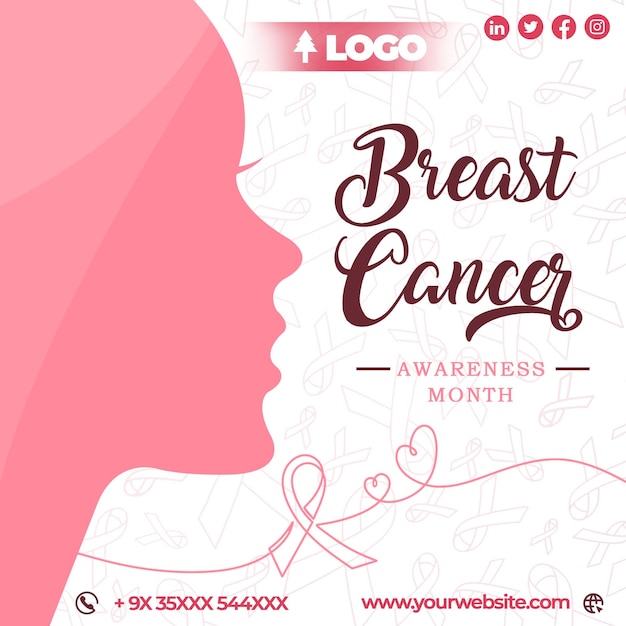This photographic image depicts a webpage with a white background adorned with pink breast cancer awareness ribbons serving as a subtle wallpaper. Central to the page is an elegant profile graphic of a woman's face, illustrated in varying shades of pink—dark, light, and pastel—showcasing her eyelashes, nose, mouth, chin, and part of her neck. 

At the top of the webpage, a prominent banner displays a red tree logo with white text. Below the graphic, the words "Breast Cancer" appear in a flowing, cursive, brown decorative font, followed by "Awareness Month" written in striking black and pink typography.

In the bottom segment of the page, there's a section dedicated to social media connections featuring circular icons for LinkedIn, Twitter, Facebook, and Instagram. These icons have red backgrounds and white logos, providing a cohesive design aesthetic. Additionally, contact information is provided at the bottom, including a phone number and a website, completing this informative and visually appealing layout focused on raising breast cancer awareness.